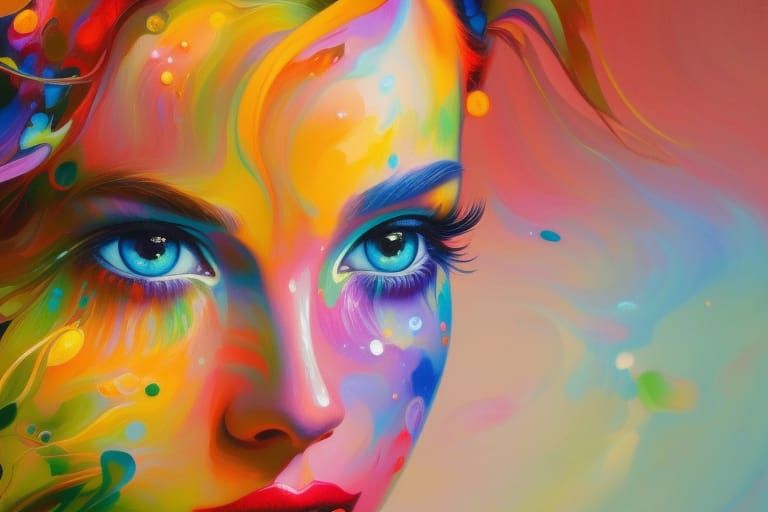This is a large, vibrant multi-color watercolor painting depicting a detailed, close-up view of a woman's face, occupying the entire left side of the canvas. The face itself is a symphony of colors, with the forehead, cheeks, and nose adorned in swirling brush strokes of yellow, pink, green, purple, and blue hues. The left cheek is illuminated with shades of yellow, red, orange, and green, while the right cheek showcases pink, blue, and purple tones. Her forehead combines these vivid colors in dynamic patterns, and the nose is primarily pink and white.

The woman's eyes are striking with large, bright blue irises, framed by meticulously detailed long black eyelashes. Her left eyebrow is brown, contrasting with a blue right eyebrow, each exhibiting fine, individual hairs. Her lips, just visible at the bottom edge of the painting, are painted with red gloss lipstick that adds a vivid touch to the composition.

On the right-hand side of the painting, the background features an abstract, swirling design in a blend of pink, blue, and green colors that merge together and transition into pale green and blue at the bottom. There are several smaller elements like green dots and interspersed dark blue swirls, adding to the complexity. Droplets of paint are visible, adding texture to the background.

The overall effect is a colorful and dynamic portrayal of a woman's face, imbued with a mixture of realism and abstract artistry, making the entire piece a bright and captivating visual experience.